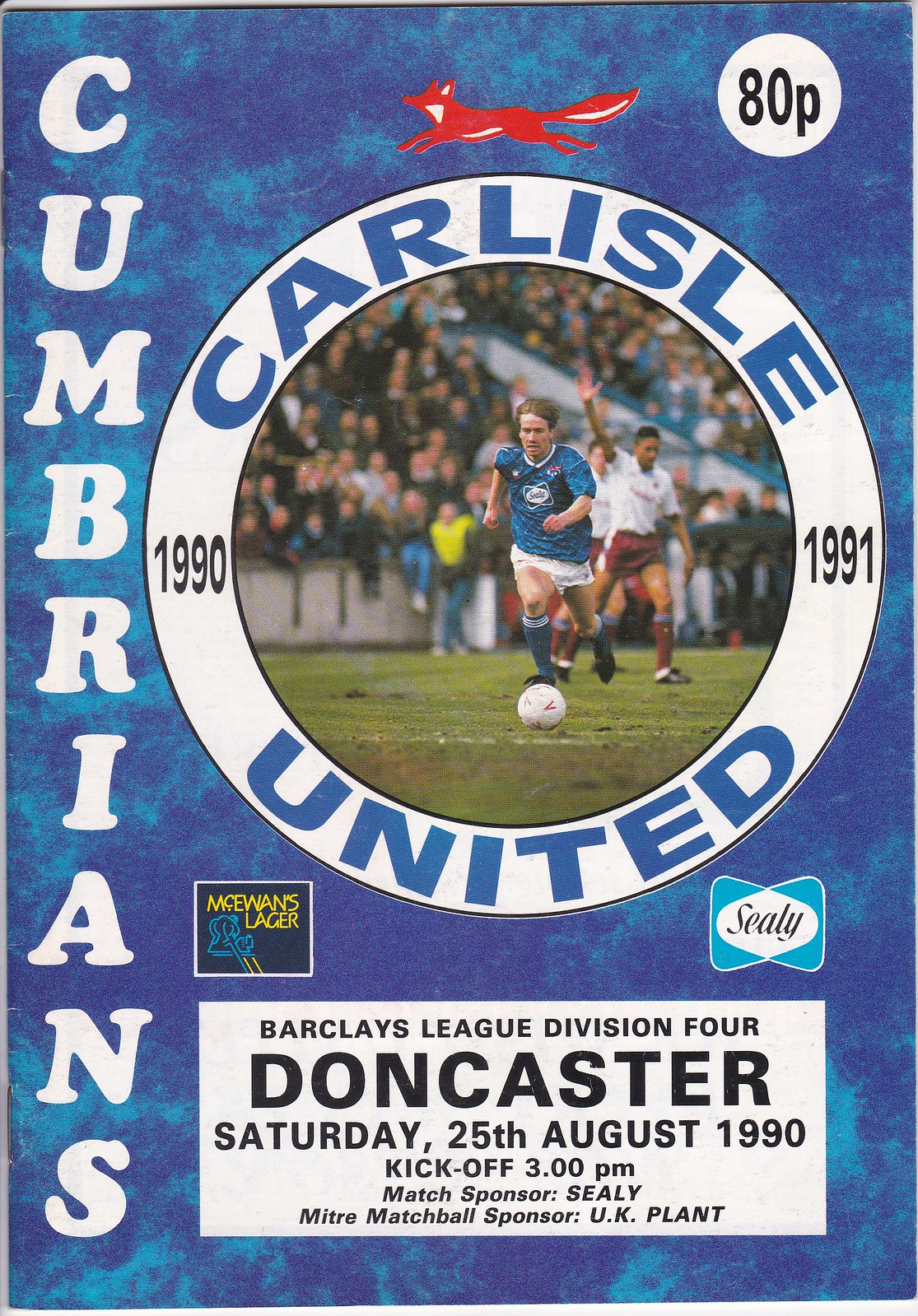This blue-toned advertisement flyer is designed to promote an upcoming soccer game in the United Kingdom, featuring vibrant imagery and detailed information. The blue background is accented with white, cloud-like splotches, lending a dynamic feel. Dominating the upper right corner is a white circle with black text reading "ADP".

The center of the flyer prominently displays an action shot of a soccer player in a blue jersey, white shorts, and blue socks, kicking a white soccer ball. This scene is set against a green field with a blurred audience in the background. Nearby, players from the opposing team are depicted in white shirts paired with maroon shorts and socks. The image is encircled by a white background, which features the text "Carlisle United 1990-91" in blue letters.

Vertical white text running down the left side spells out "CUMBRIANS" in bold capital letters. Just above the center image, there's a portrait of a red fox, symbolizing the team's emblem. Beneath this emblem, advertisements are strategically placed, including the Sealy logo in black letters on a white background outlined in blue, and the McEwan's Lager logo in yellow on a dark blue or black background.

At the bottom of the flyer, a white rectangle contains crucial event details in black capital letters: "Barclays League Division 4, Doncaster, Saturday, 25th August 1990, kickoff 3 pm". It also lists sponsors, including Sealy, Mitre, and UK Plant, making this flyer both informative and visually engaging.